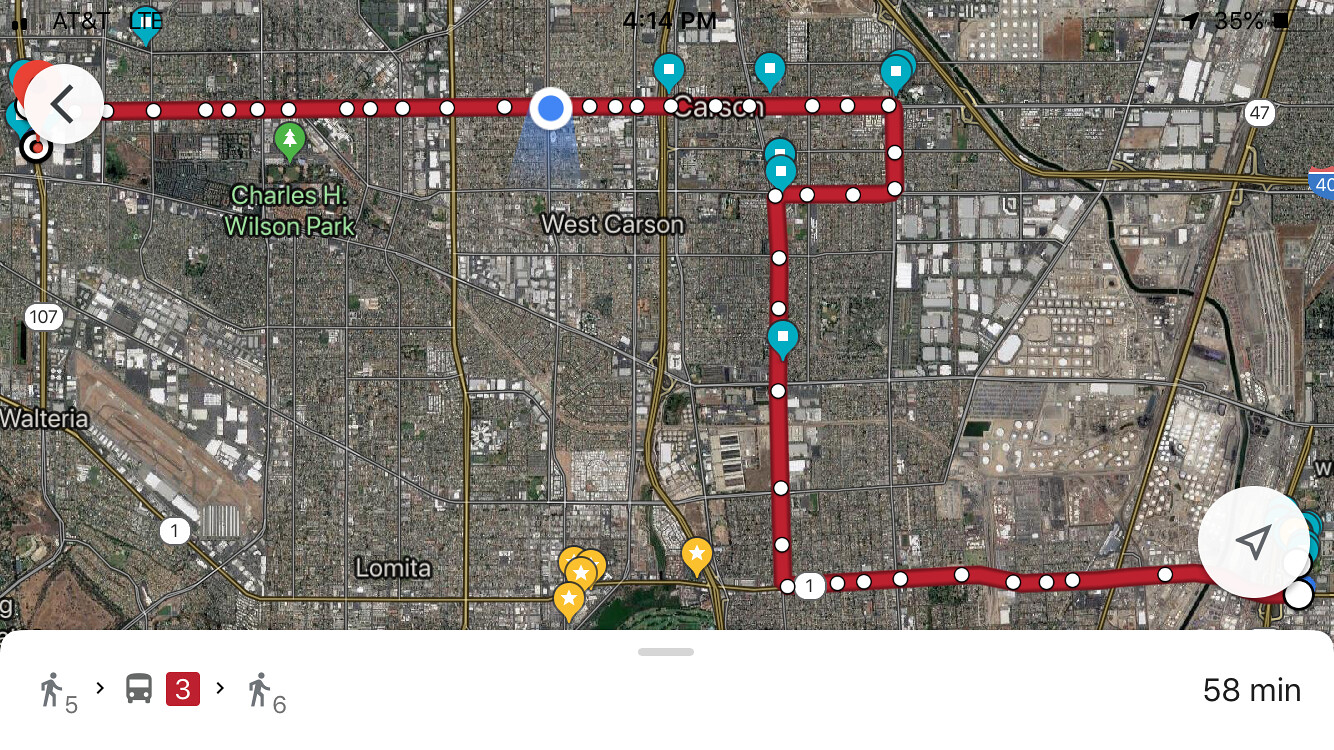The image depicts a detailed map of New York City, specifically highlighting various routes and landmarks. Notable locations labeled on the map include Alameda, West Charleston, Charleston H. Wilson Park, among others. A red line traces a specific route on the map that extends from one point to another, covering an estimated travel time of about an hour. The journey appears to include a walking segment of approximately five minutes, followed by a bus ride involving routes 3 and 6. The visual representation strongly resembles the interface of Google Maps, providing a clear and organized layout of the described travel path.